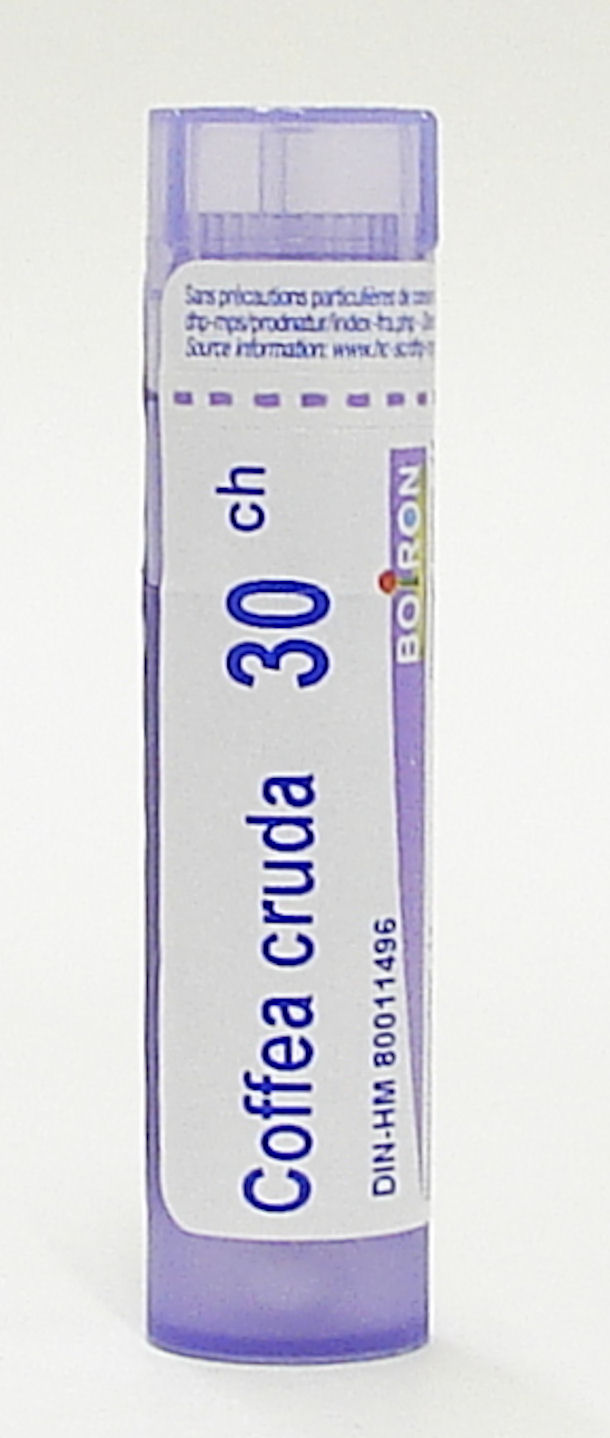The image features a tall, vertical, rectangular product with a gray background. The product, a small clear plastic bottle with a purple tint, is designed for easy portability and appears to be user-friendly. Dominating the bottle's front is a white label with vertical text reading "Coffea Cruda" in a thin, blue font. Adjacent to the text is a prominent blue number "30," and above it, slightly to the left, the letters "CH." Below "Coffea Cruda," a series of letters and numbers "DIN-HM 800-11496" is visible, indicating the health identification number. To the right, in smaller white font on a light purple background, is the word "Boiron." This bottle, topped with a plastic screw-off cap for secure closure, is intended for relief of chronic pain and nerve sensitivity. The packaging suggests practicality, suitable for carrying in a pocket or purse.